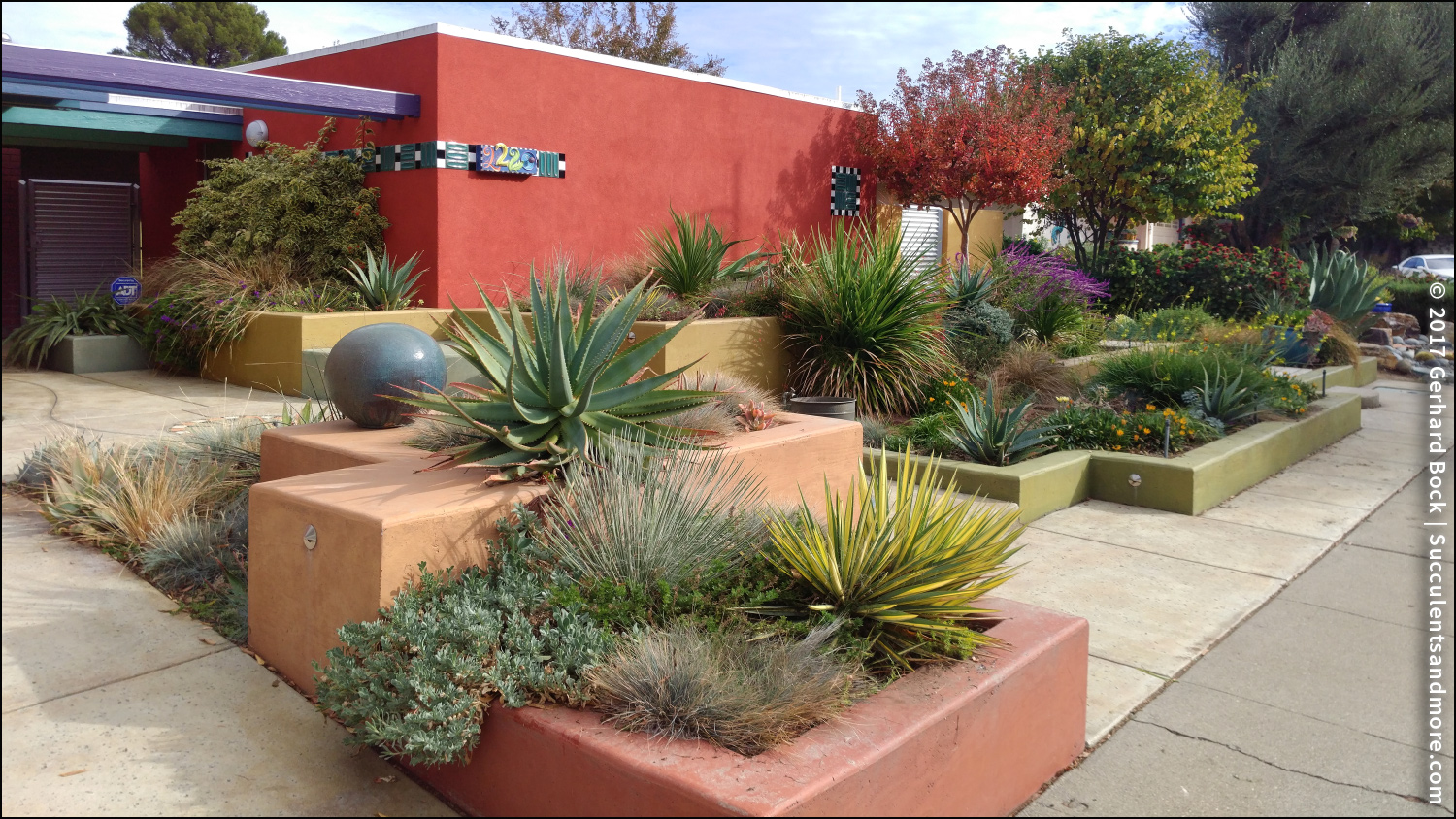The photograph captures the exterior of a one-story, salmon pink stucco building adorned with the number "222" on its corner, complemented by an adjacent blue ADT security sign. A distinctive purple beam juts out from the left side of the building, which also features a metal doorway. In front of the building spans a sidewalk bordered by square cement planters brimming with a diverse array of desert vegetation, including various cacti and colorful flowering plants in shades of purple and yellow. The planters present a vibrant mosaic of colors such as red, orange, and green. The scene is enveloped by the backdrop of a cloudy blue sky and some distant trees, adding to the lively yet serene atmosphere.